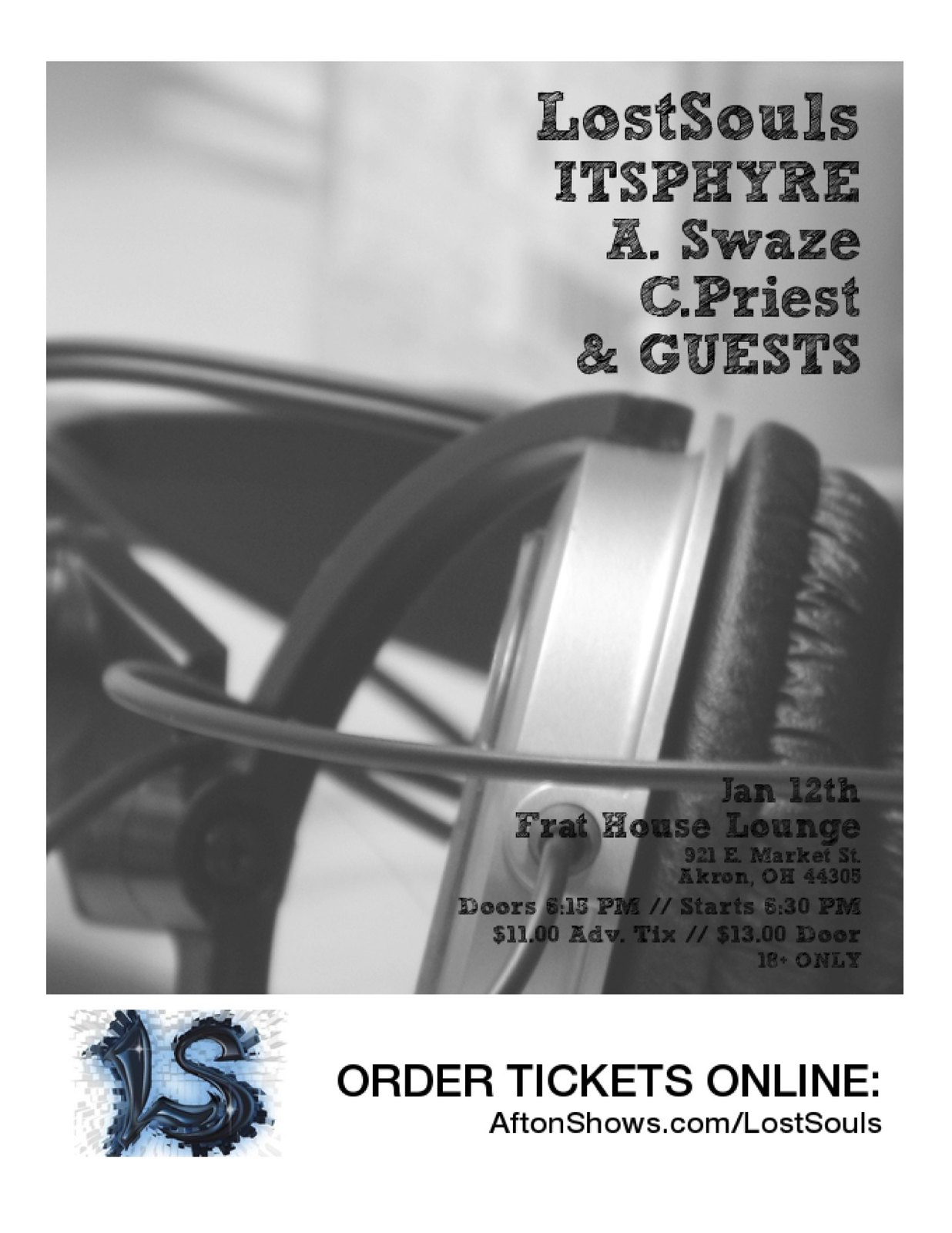This portrait-oriented black-and-white image serves as an advertisement for a musical event. The dominant visual is a close-up photograph of a single over-ear headphone, intricately wrapped with its own wires, emphasizing the texture and form of the audio equipment. In the top right corner, bold black text declares "Lost Souls," with the capital 'L' and 'S' catching the eye, alongside additional performers including "It's Fire, A. Sways, C. Priest, and Guests."

At the bottom right corner, detailed event information is provided: "January 12th, Frat House Lounge, 921 East Market Street, Akron, Ohio, 44305, doors open at 6:15 PM, starts at 5:30 PM, $11 advanced tickets, $13 at the door, 18+ only." Below this, a white horizontal border spans the width of the image, containing a blue and black abstract logo featuring the initials 'LS,' reminiscent of spilled ink. To the logo's right, text directs viewers to "Order Tickets Online: aftonshows.com/lostsouls," seamlessly integrating photography with graphic design.